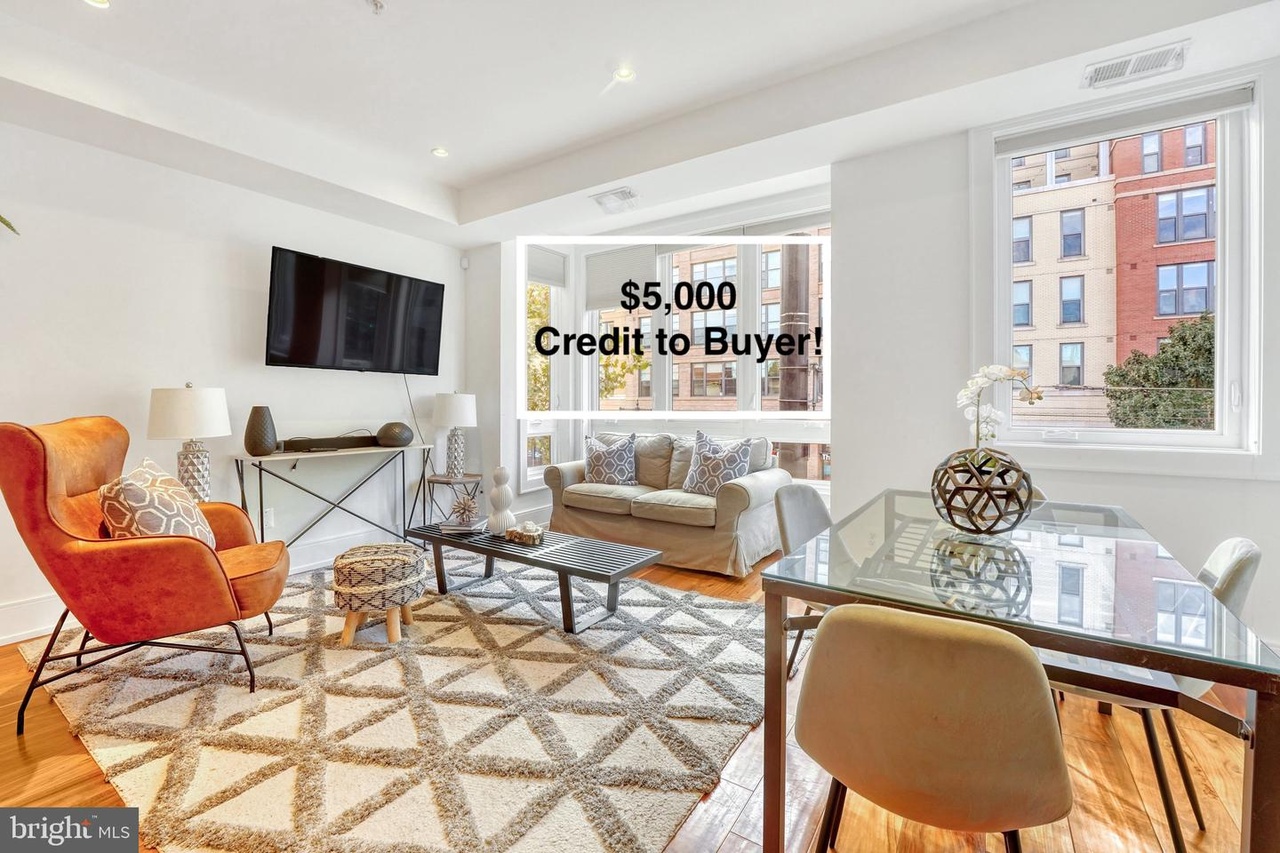This image is a horizontal color photograph showcasing a modern and elegantly-designed apartment living room as part of an advertisement for Bright MLS. In the lower left-hand corner, "Bright MLS" is displayed in small white letters within a dark gray box. The main promotional message, "$5,000 credit to buyer", is prominently positioned in black text across the top center of the photograph.

The room is strikingly well-lit, featuring natural light streaming in through a large picture window located behind a low, modern couch in the center of the image. The bright, airy ambiance is complemented by white walls and a ceiling that enhance the spacious feel of the room.

On the right side, a glass tabletop adds a touch of sophistication while reflecting part of the room's decor, including a globe. Adjacent to the glass table is a smaller, square window through which several apartment buildings are visible.

The furnishings underscore a contemporary aesthetic: a triangular-patterned shag rug anchors the space, centered by a small, sleek, metal coffee table. An eye-catching orange low chair adds a pop of color to the left of the image. To the right, a widescreen TV is mounted on the wall, situated above a long white table adorned with two elaborate table lamps and various decorative objects.

Finishing touches such as two plush pillows on the couch and the overall meticulous arrangement of decor elements enhance the room's inviting and stylish atmosphere.